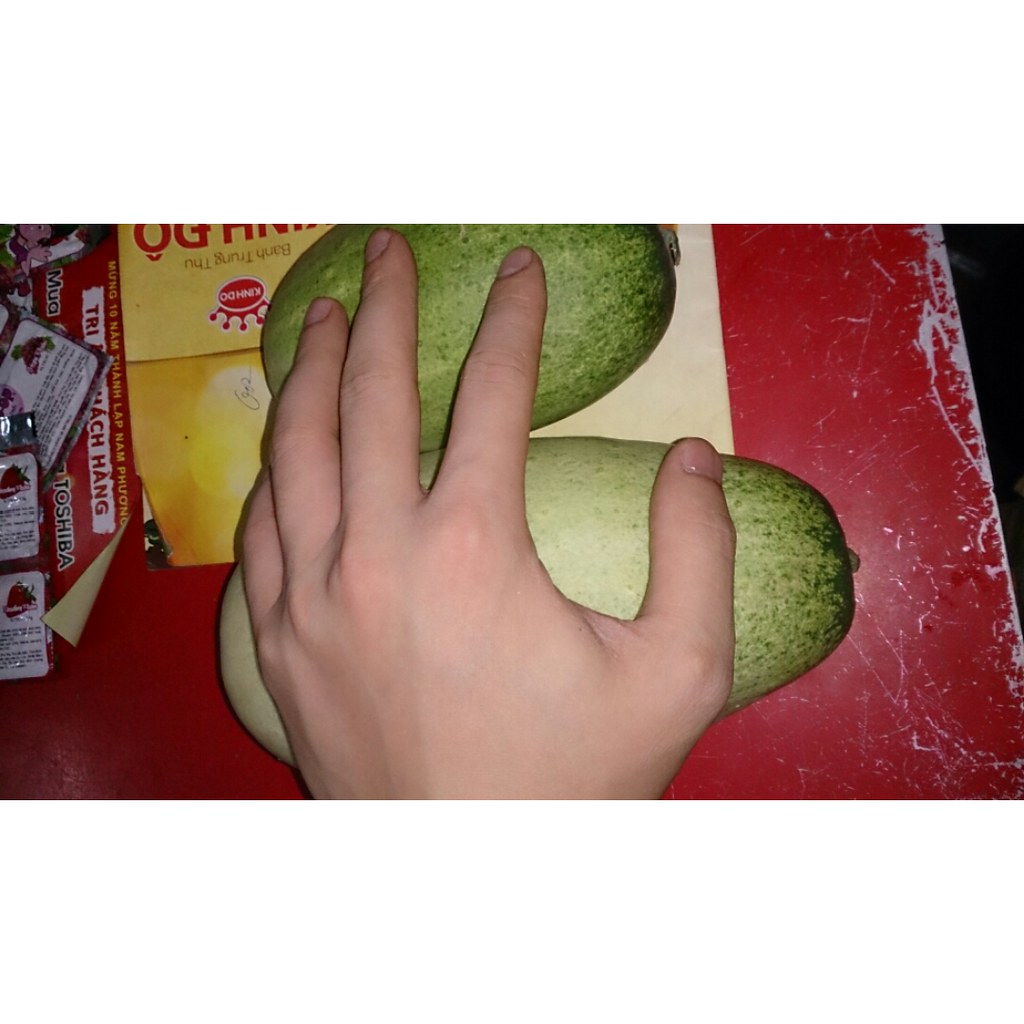In this image, a person's left hand is positioned prominently in the foreground, with their wrist up and thumb oriented to the right, resting on two oval-shaped fruits or vegetables that are larger than avocados. These items have a unique texture and coloring similar to small watermelons, featuring dark green and speckled green surfaces interspersed with patches of yellowish light green. The red countertop beneath them exhibits signs of wear, with areas where the paint has been scraped away, revealing a silver color underneath, especially noticeable on the edge. To the left of the image, there are several small packets, including one with a red and white label that reads "TOSHIBA" in vertical black text. Nearby, a plastic packet with a red and cream white label displays the partially visible words "TRY" and "HANG". Additionally, there is a yellow advertisement with red designs and white text, featuring a red crown and foreign language script saying "KINHDU, PANTRUDU". The presence of these varied elements lends a cluttered yet vivid scene, enhanced by the detailed textures and colors.